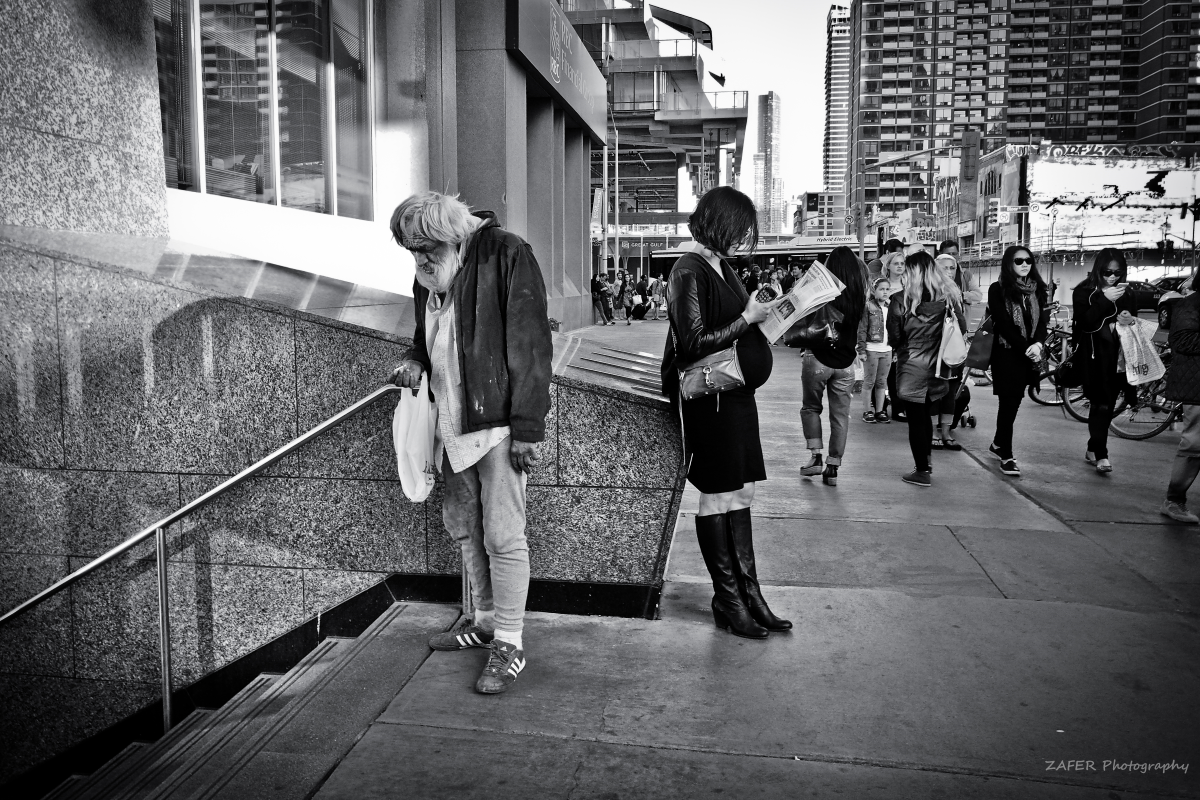In this black and white photograph taken in a bustling city center, an old man, appearing homeless with his disheveled hair and worn-out, dirty clothes, stands at the top of a staircase that seemingly leads to a subway tunnel. He's holding a white plastic bag and looks forlornly down the steps. To his right, leaning against the building's protruding structure, is a well-dressed woman with cropped black hair, wearing high black boots and a skirt. She holds a newspaper and possibly a phone in her hand, seemingly engrossed in her reading. The busy city scene is further accentuated by numerous people in the background, mostly women, walking in various directions; some are engrossed in their phones while others move purposefully along the sidewalk. In the distant background, an apartment building or perhaps condos, can be observed, adding depth to the urban environment. The photograph is titled "The Fair Photography," inscribed at the bottom.